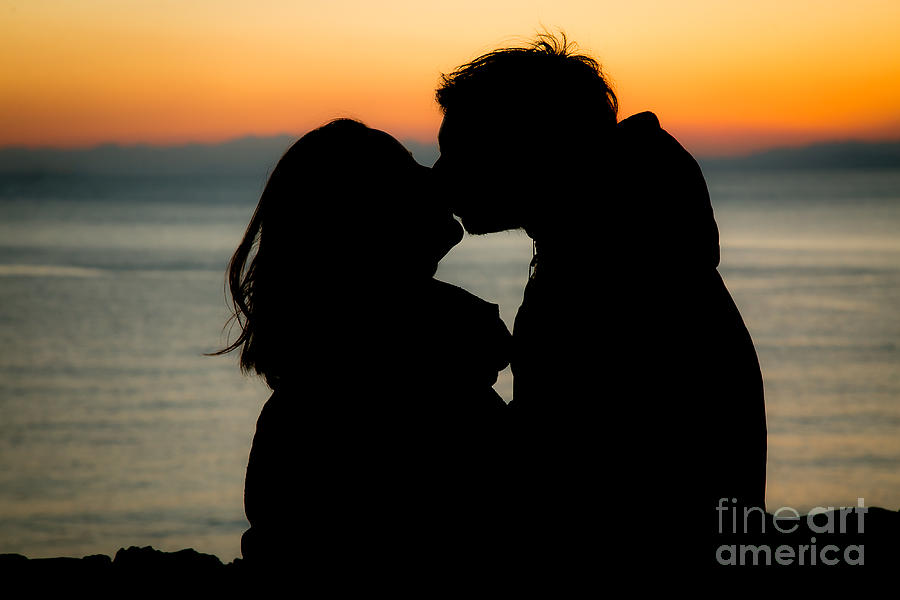This photograph, possibly featured on the Fine Art America website, captures a tender moment of two people kissing, silhouetted against a stunning sunset. Positioned in the lower right corner, the watermark "Fine Art America" is visible. The image showcases a beach setting with ocean waves, framed by distant hills or perhaps another island with rocky formations. The couple, cropped at the waist, are dressed in jackets, suggesting a chilly yet romantic atmosphere. She has short brown hair, while his hair is also short. The dramatic sky transitions from deep red and pink near the horizon to vibrant orange and yellow, gradually blending into subtle hints of blue. The overall composition highlights the couple's embrace, set against the blurred yet serene expanse of the ocean and the striking sunset colors, creating an evocative silhouette art piece.